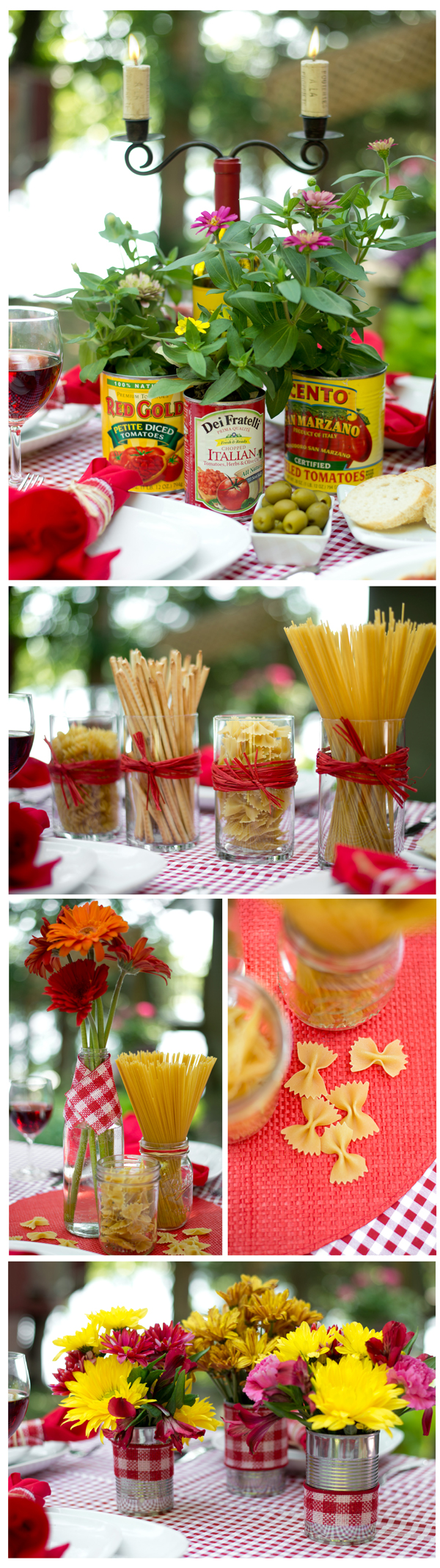This long vertical montage features five images, each detailing an eclectic mix of Italian food and creatively decorated table settings, seemingly captured in an outdoor setting. The topmost panel showcases three brands of diced or chopped tomatoes cans, including 'Red Gold' and 'Cento,' repurposed as vases for vibrant flowers. These cans, adorned with gold and checkered ribbons, are part of a lively tablescape that includes a white dish of green olives, a glass of wine, and untouched place settings with bruschetta bread and napkins. 

Below this, the next image highlights four different-sized clear glass jars wrapped in red string, each filled with various forms of raw pasta. The subsequent pair of images displays more of this setup; on the left, a jar of pasta sits beside a bouquet of flowers, while on the right, bowtie and angel hair pasta rest on a red tablecloth. 

The final panel at the bottom presents additional cans turned floral vases, these with their labels removed and wrapped in black-and-white checkered ribbon, all positioned on a table covered with a red checkered tablecloth, completing the rustic yet elegant theme.